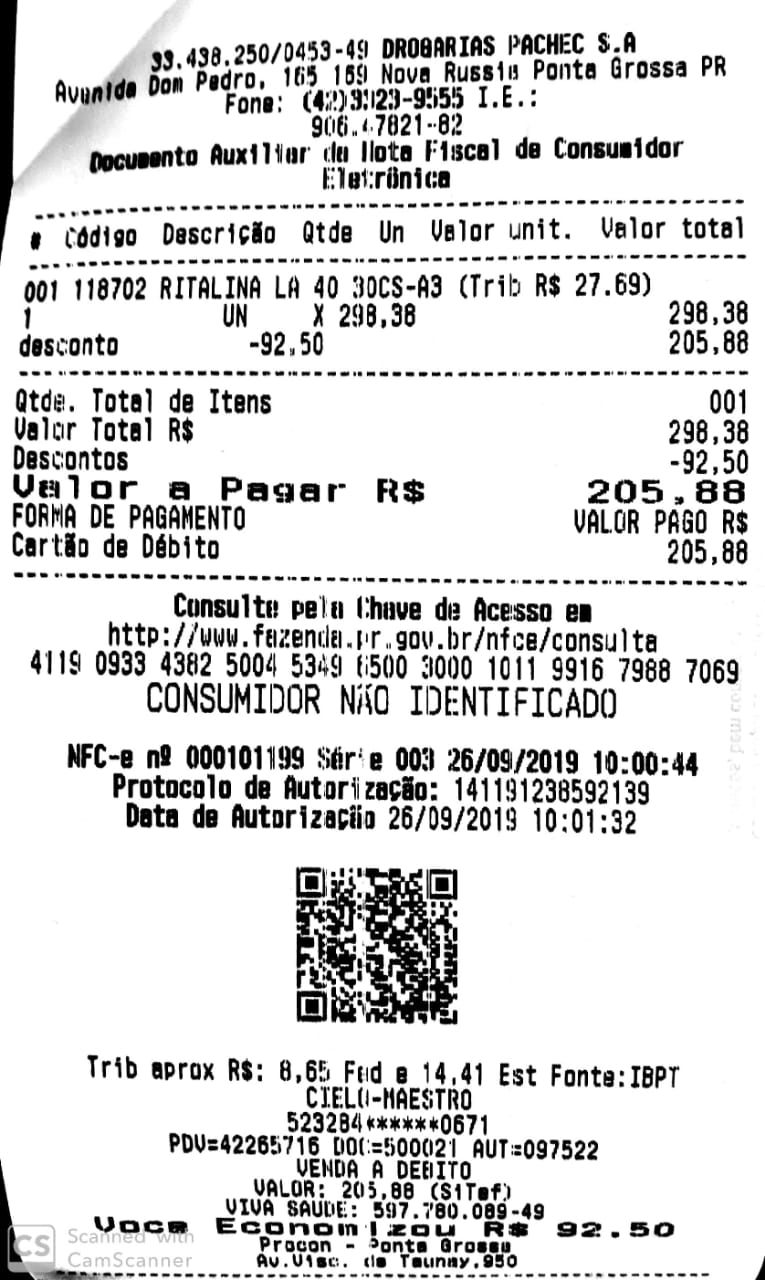A portrait-oriented receipt printed on white paper with black text and numbers displayed in Spanish. The receipt features a QR code at the bottom, and the total amount is $205.88. The timestamp on the receipt reads 10:01:32, dated September 26, 2019. It details the purchase of a single item initially priced at $298.38, which received a discount of $92.50.